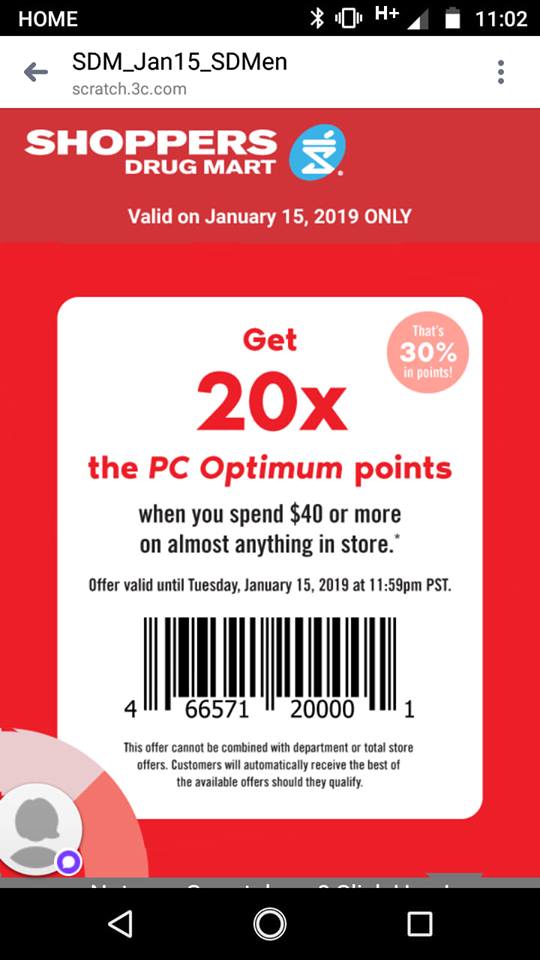**Detailed Descriptive Caption:**

The image is a screenshot of a smartphone displaying an advertisement. At the top of the screen, a black bar features various icons in white: a Bluetooth icon, a signal strength icon, and battery status indicators. The time displayed is 11:02. On the top-left corner, the word "Home" is displayed. Below this black bar is a white bar containing the text "sdm-jan15-sdmen," alongside a left-pointing arrow for navigating back to the previous screen and three vertically stacked dots on the right side for additional options.

The main content of the ad dominates the majority of the screen space with a vibrant red background. At the top of this red section, there is a darker red bar with the text "Shoppers Drug Mart" in white letters. To the right, within a blue oval, there's an icon resembling a mortar and pestle, accompanied by the text "Valid on January 15th, 2019 only."

Beneath this, a slightly lighter red area encloses a white square. Inside the white square, the text "Get 20x the PC Optimum points" is written in red. A nearby circle indicates that this reward equates to "30% in points." This offer is valid when spending "$40 or more on almost anything in-store," with an asterisk next to this statement hinting at further terms and conditions. The validity of the offer extends until Tuesday, January 15th, 2019, at 11:59 PM PST. A large scannable UPC barcode is prominently displayed for cashier use.

In the bottom-left corner of the screen, there's an icon of a person, likely representing the user's account where they can upload their avatar. Finally, at the very bottom of the screen, a black navigation bar includes typical app buttons such as the home and back buttons.